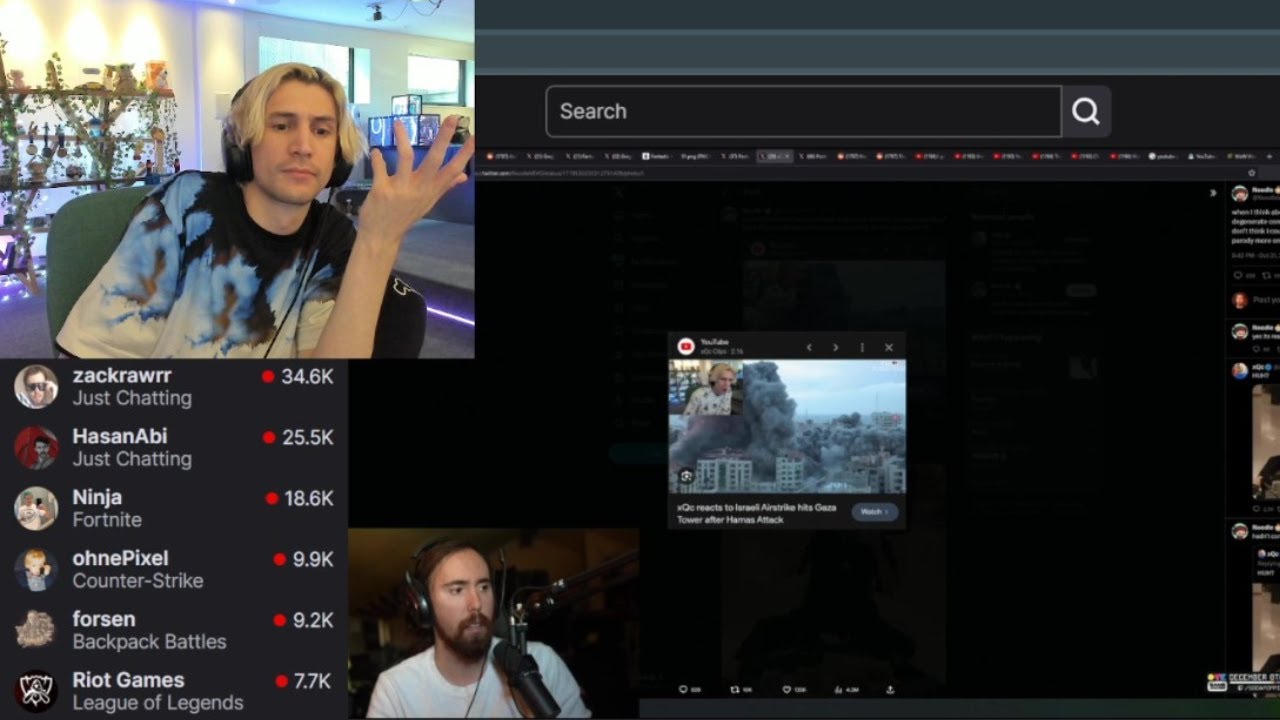The image features a collage of popular streamers in a multi-streaming layout. In the top left corner, a box contains the streamer XQC, who is wearing a blue and white cloud-patterned shirt and headphones. His left hand is raised and tilted slightly. Below XQC's box, a smaller box displays Asmongold, dressed in a white shirt, also wearing headphones and speaking into a microphone attached to a black boom arm.

To the left of these boxes are additional streamer profiles with their viewer counts. These include Zack Rahr with 34.6K viewers, Hasan Abi with 25.5K viewers, Ninja with 18.6K viewers, OnePixel with 9.9K viewers, Forsen with 9.2K viewers, and Riot Games with 7.7K viewers. Beneath each name, the games they are currently playing are listed.

On the right-hand side of the image is a black search bar and an open tab, as well as a thumbnail featuring XQC reacting to a video showing buildings with a large explosion.